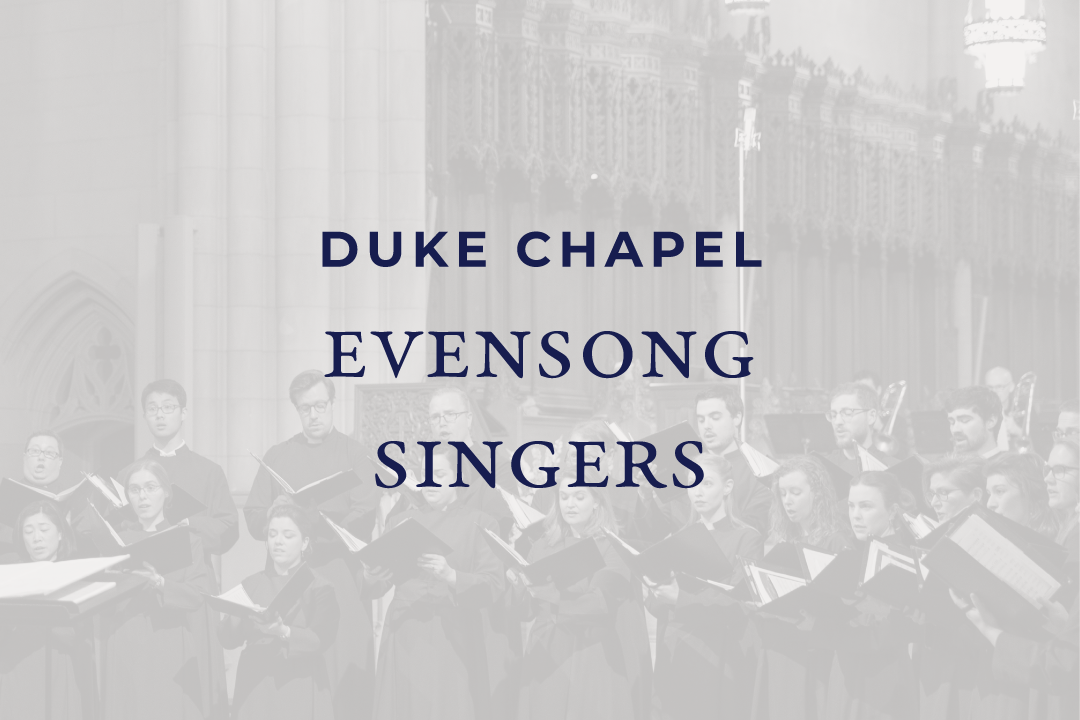This black-and-white photo features a large choir, composed of both male and female members, dressed in traditional performance gowns with distinctive white collar inserts and white triangle designs running from shoulder to chest. The choir members, some of whom appear to be priests, hold music sheets while others play instruments like trumpets, and they are all facing towards the left. In the backdrop, you can see what appears to be the interior of Duke Chapel, with visible walls and a chandelier in the upper right corner. The background also includes rows of confession stalls and an arch, indicative of a chapel setting. The image is slightly grayed out, giving it a blurred effect, and overlaid with the black text "Duke Chapel Evensong Singers." The words "Duke" and "Chapel" are written in a thicker font, while "Evensong Singers" appears in a thinner, larger font, both in a dark blue color.